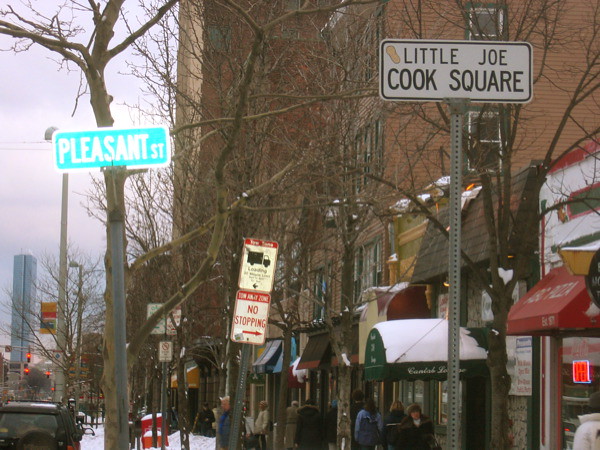A winter street scene titled “Little Joe Cook Square” showcases a snow-dusted urban environment. Barren trees line the street, signifying the season's cold embrace. Prominent signs in the foreground include a green street sign for Pleasant Street, a No Stopping sign, and a truck loading zone sign with partially obscured text. To the right, a series of smaller shops line the road, characterized by snow-covered roofs, against the backdrop of a larger, partially obscured building ensconced by numerous trees. The sidewalk and distant buildings are lightly blanketed in snow, completing this tranquil winter tableau.